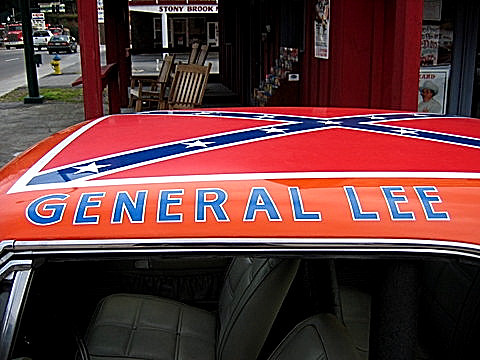In this vibrant close-up photo taken outdoors, we see the iconic General Lee car from the "Dukes of Hazzard." The car features a deep orange exterior with the Confederate battle flag prominently displayed on the roof. The flag is depicted as a red rectangle bordered in white with a blue X overlayed with white stars. The words "General Lee" are written in blue on the top. Through the open driver's side window, the car's interior is visible, showcasing black leather seats. The photo's background reveals an old-fashioned store with a reddish wooden facade, complete with wood rocking chairs and a magazine stand out front. Part of the road is visible in the upper left corner, where traffic passes by. Additionally, a yellow fire hydrant can be seen near the road. Further in the distance, another store sign reads "Stony Brook" in white text on a black background, adding to the quaint, nostalgic ambiance of the scene.